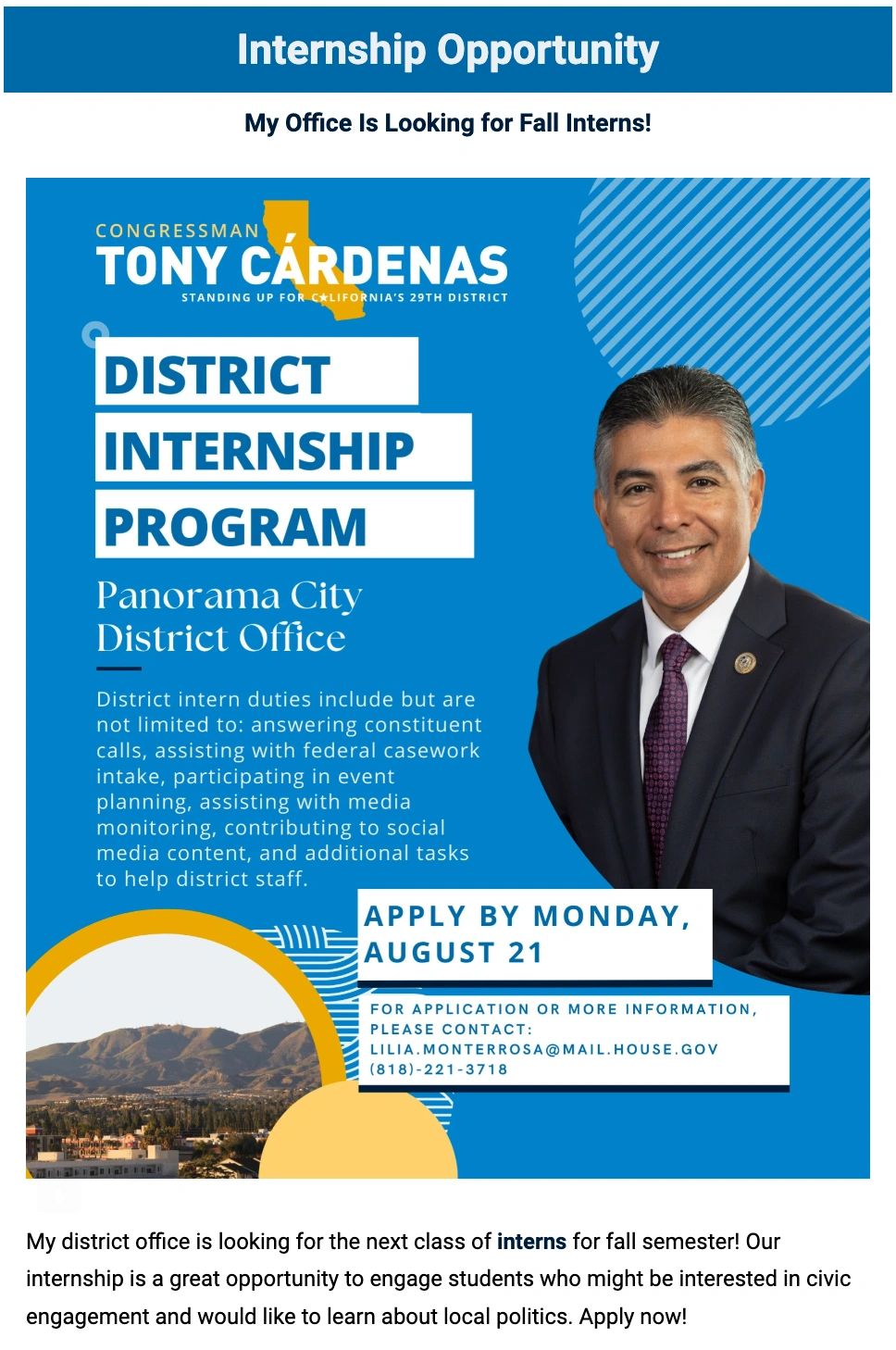The flyer advertises an internship opportunity for Congressman Tony Cardenas of California's 29th District. It prominently features a large, mostly blue background with white text, announcing, "Internship Opportunity: My office is looking for fall interns." The central image is a photograph of Congressman Tony Cardenas positioned on the middle right. He has gray hair on the sides and black hair on top, and is wearing a black suit, white shirt, and purple tie. The flyer describes the internship as a valuable experience for students interested in civic engagement and local politics. Additional text includes, "District Internship Program," "Panorama City District Office," "Apply by Monday, August 21st," and for more information, instructions to contact the office are provided. A small image of the California state outline in yellow and a photograph of the Panorama City district showing mountains, houses, trees, and clouds are located at the bottom left. The flyer incorporates a variety of colors, including lighter and darker shades of blue, tan, black, white, purple, burgundy, and dark orange.